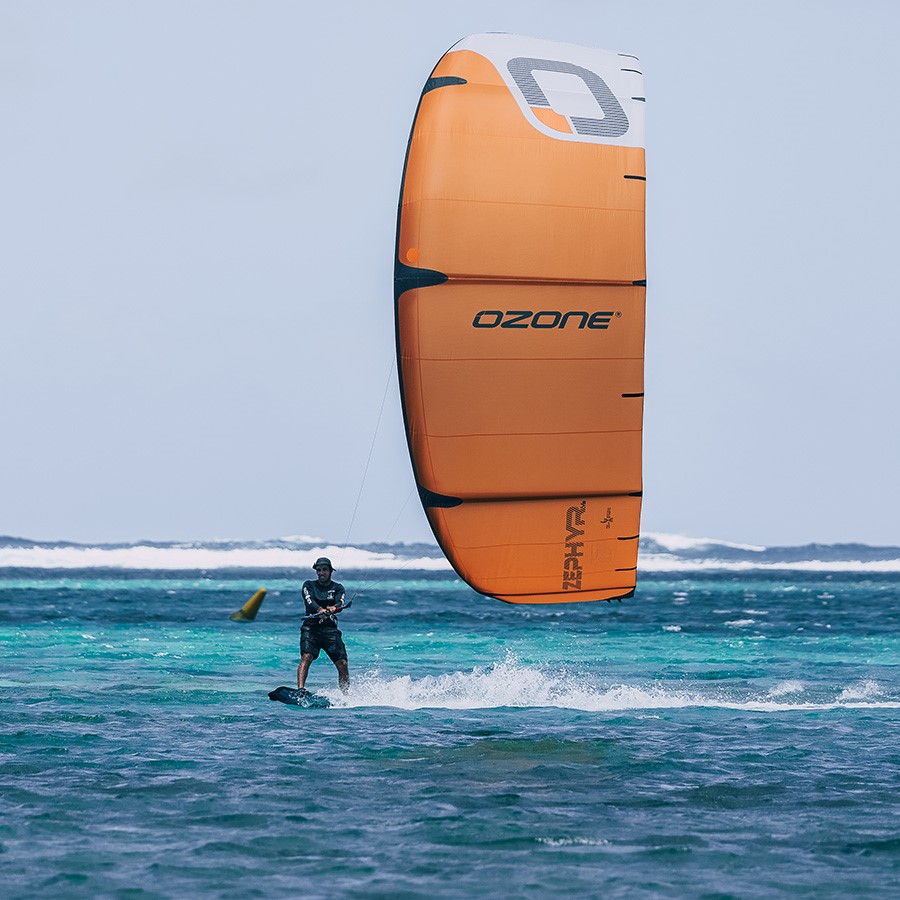The image depicts a man engaged in kite surfing over crystal blue ocean water, which features a mix of light blue, greenish, and darker blue hues. The sky above is a cloudy gray, creating a stark contrast with the vibrant scene below. The kite surfer, wearing bathing suit shorts, a water shirt, and a hat, firmly grips the lines of an enormous orange kite behind him. The kite is adorned with the brand logo "Ozone" prominently displayed in the center, accompanied by the word "Zephyr" at the bottom. The logo also includes a large circle symbol with the bottom left segment highlighted in orange and bordered in black, adding a distinctive mark to the vividly hued kite. The overall composition captures the dynamic energy of kite surfing with strikingly clear water and a vast, slightly ominous sky.